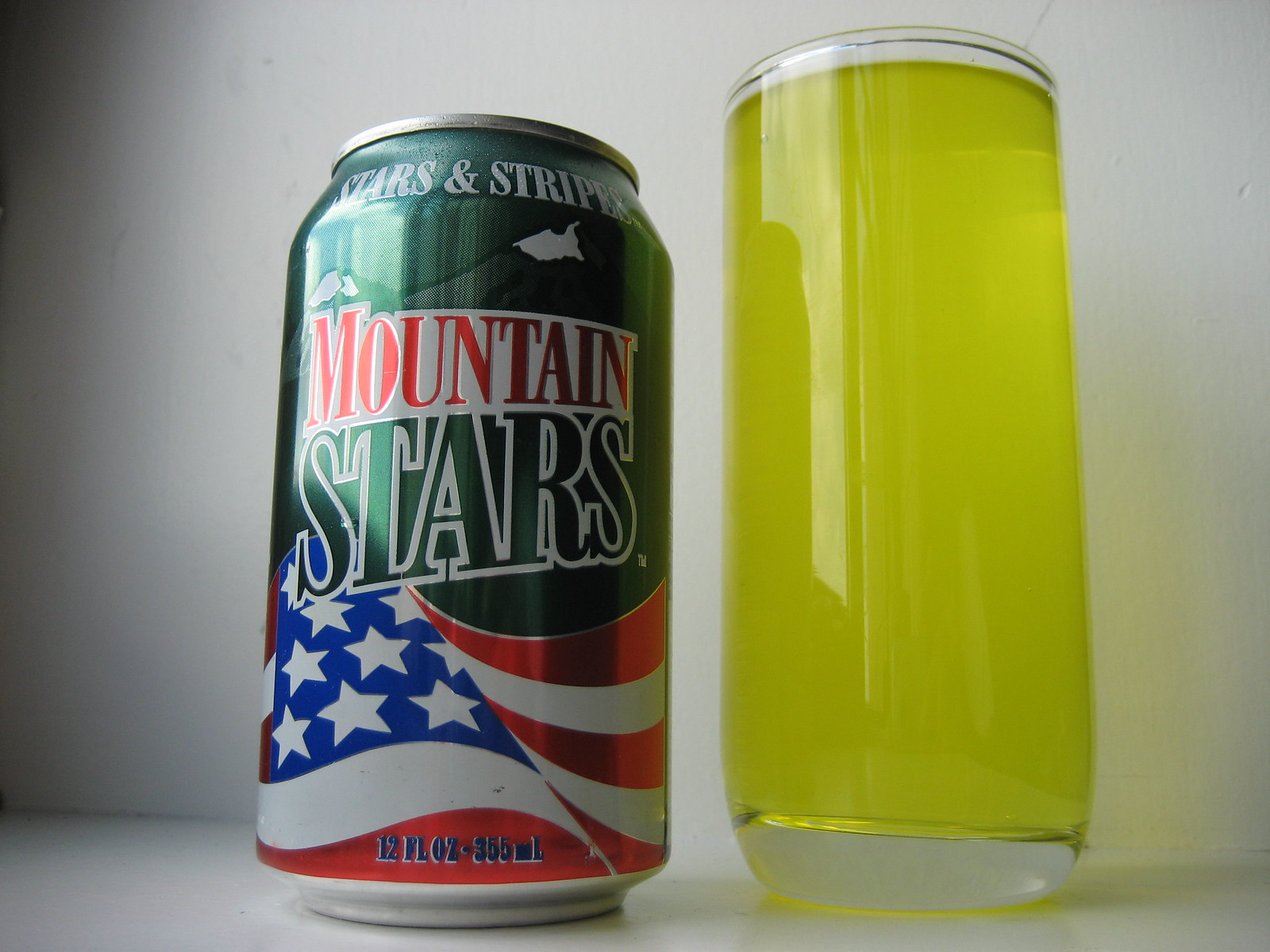The professionally photographed image captures a beverage setup against a pure white background, typically used for product advertisements. On the left side stands an aluminum can, prominently displaying the text "Stars and Stripes" at the top followed by "Mountain Stars". The word "Mountain" appears on a white banner in bold red letters, contrasting with the embedded "Stars" in white, outlined against the green background of the can. A rippled American flag embellishes the lower part of the can, which is labeled with a capacity of "12 fluid ounces" or "355 milliliters". To the right of the can sits a tall cylindrical glass jar, marginally taller than the can itself, filled to the brim with a yellowish-green liquid reminiscent of Mountain Dew. The entire setup is positioned on a white shelf or counter, with a subtle black vignette on the left side adding depth to the scene. The minimalist background and precise arrangement emphasize the vivid colors and details of the can and its contents, making it likely intended for a food or beverage advertisement.